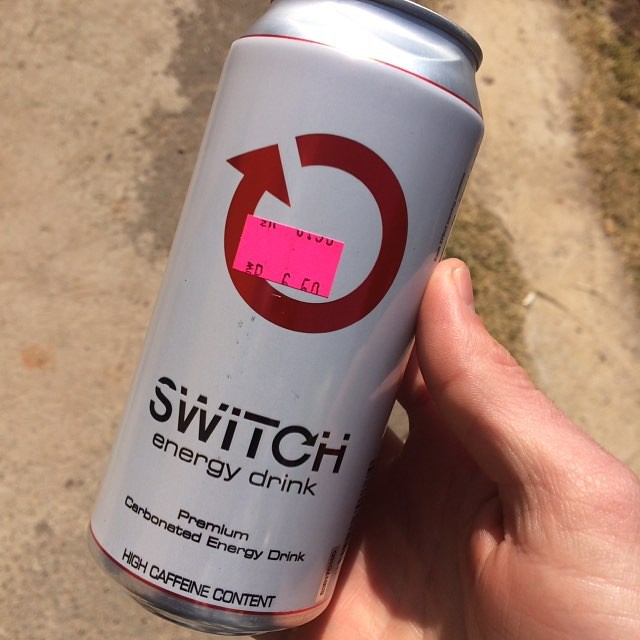In this detailed image, a hand is prominently holding a canned beverage. The can features a sleek silver or gray design. Notably, there is a circular symbol with an arrow at the end, adding a unique touch to its appearance. The upper half of the can bears a pink tag, hinting that the product might have been on sale, though the details on the tag are not fully legible. 

The brand name "SWITCH" is clearly displayed in bold black letters towards the lower part of the can. The lettering style includes a distinctive "C" with a circle symbol, giving it a unique identity. Beneath the brand name, in black letters, the product is labeled "ENERGY DRINK." Further down, in even smaller black lettering, it reads "PREMIUM CARBONATED ENERGY DRINK."

At the very bottom of the can, in small block capital letters, is a warning that states "HIGH CAFFEINE CONTENT." The can is held securely in the palm of a person's hand, as they present it directly to the camera lens, ensuring all the details are visible.